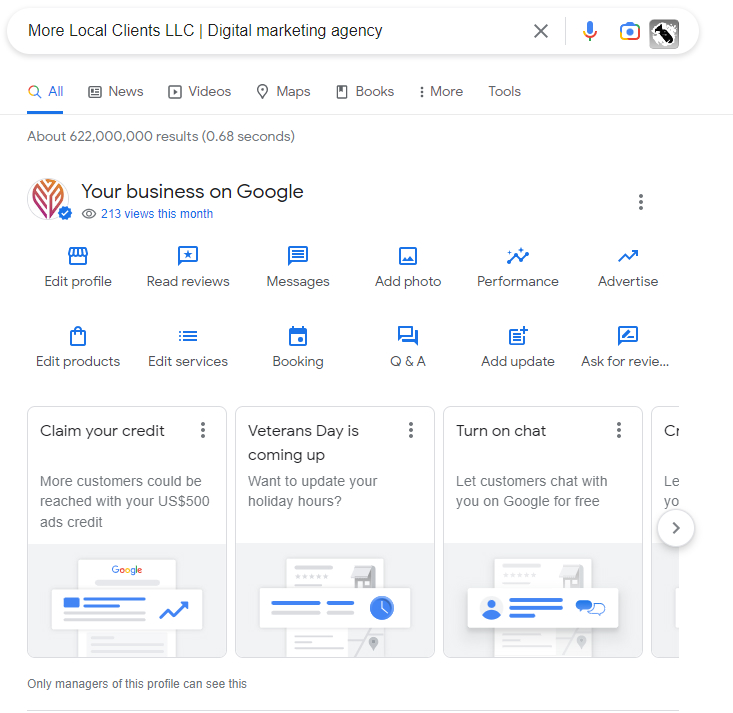A detailed, cleaned-up caption for the image could be:

"This image depicts a personalized business page for a digital marketing agency named 'More Local Clients, LLC,' managed through Google. Displaying their Google Business profile, the page achieved 213 views this month. The Google search results show approximately 622 million results in 0.68 seconds. At the top, a navigation menu offers options like All, News, Videos, Maps, Books, More, and Tools. The interactive section of the business profile includes various management options: Edit Profile, Read Reviews, Messages, Add Photo, Performance, Advertise, Edit Products, Edit Service, Booking, Q&A, Add Update, and Additional Requests. The lower part of the screen features three noticeable promotional boxes and a fourth partially visible one. The promotions include: 'Clean Your Credit,' 'Gain More Customers with a $500 Google Ads Credit,' 'Veteran's Day is Coming; Update Your Holiday Hours,' and an option to 'Turn on Chat to Communicate with Customers for Free on Google.' Additionally, there’s an unusual element in the search bar displaying a nuclear bomb icon, alongside standard microphone and camera icons."